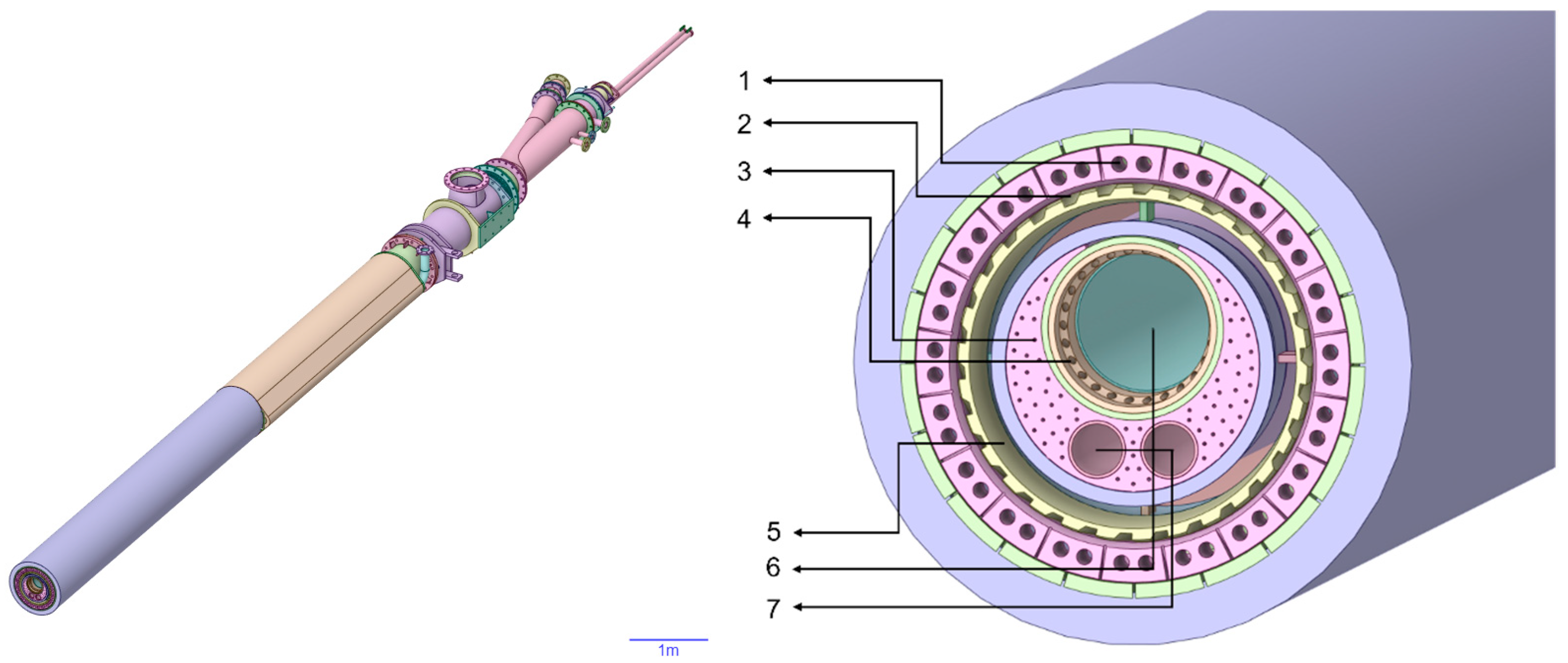The illustration showcases a flat, colorful depiction that appears to draw inspiration from design tools such as Illustrator, Affinity, Procreate, Clip Studio Paint, or After Effects. It features a long, cylindrical structure resembling either metal or plastic piping. The cylindrical pipe exhibits a repeating color pattern from left to right—purple, brown, purple, green, purple, pink, green, and purple. Various parts like offset pipes and valves are attached, creating a complex design similar to a cross-section of a mechanical or electrical system.

To the right of this cylindrical structure, there is a detailed diagram highlighting a cross-sectional view of the cylinder’s diameter. This cross-section reveals multiple layers: an outer purple ring, followed by green, pink, green, and blue rings. Within the innermost blue ring, there's a green circle at the top flanked by two smaller pink circles at the bottom. Lines extend from these sections, each marked with numbers 1 through 7, but without accompanying explanatory text. The image is highly detailed, showing intricate layering and connections, designed to visually dissect and label the different sections of the cylindrical piping or cable system.